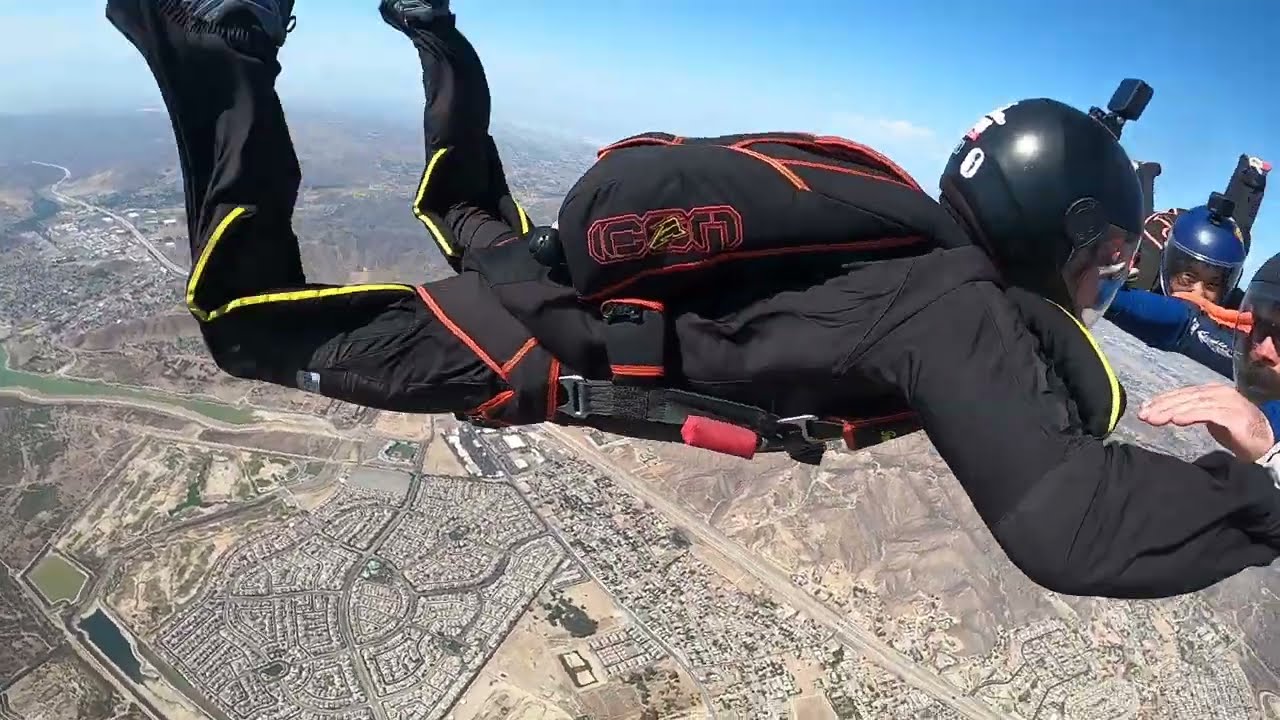The photograph captures a thrilling skydiving scene under a clear blue sky. The central figure, garbed in a black tracksuit with yellow trim, sports a black helmet equipped with a clear visor and an action camera on top. A packed black parachute with orange trim is strapped to their back. They are flanked by other skydivers holding onto their arms: to their right, only the hand of an unseen individual is visible, while to their left, a skydiver in a blue helmet and jacket, also with a camera on their helmet, is clearly seen. Below, the landscape reveals a suburban area with numerous grids of housing tracts amidst an arid environment, interrupted only by a thin river running through the left side of the image. Mountains and rocks add a rugged texture to the backdrop, enhancing the sense of altitude and adventure.